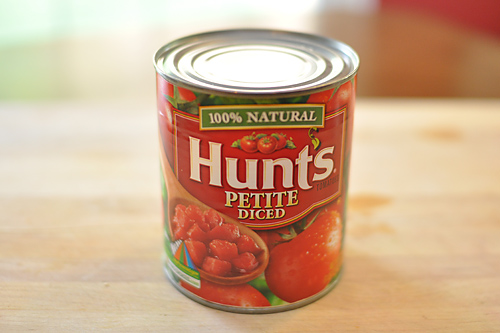A photograph captures a can of Hunt's Petite Diced Tomatoes sitting on a light-colored wooden surface, which could be a countertop, butcher block, or cutting board. The wood grain extends into the background, suggesting it might be a countertop. The can's silver lid glints under soft, white ambient light. The label is a vibrant mix of red, green, white, and yellow, featuring a green rectangle with a yellow border that states "100% natural." The label also displays images of diced tomatoes, a whole tomato, and a wooden spoon laden with the product against a red backdrop. The scene is subtly accented with blurred hints of red and green in the background, adding to the overall warmth of the image.